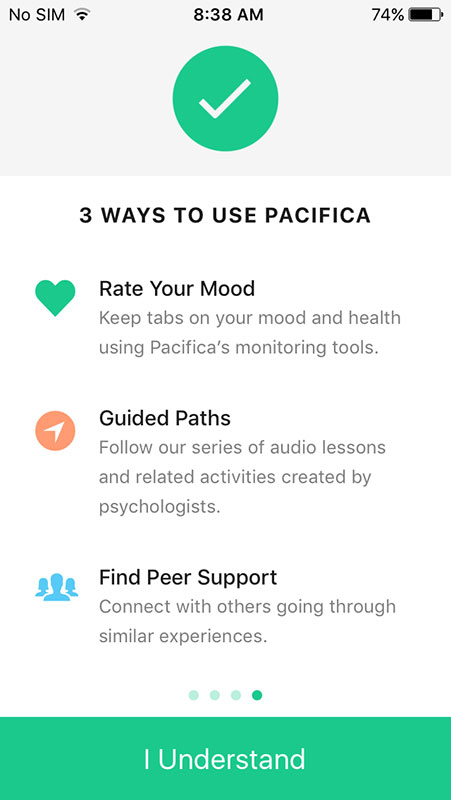In the upper right corner of the image, the battery life of the phone is displayed at 74%. Centered at the top is the time, showing 8:38 AM, and on the left, "NO SIM" is written in all capital letters next to an icon of a speaker. Below, in a green circle, there is a white checkmark.

The main content of the image introduces three ways to use Pacifica. 

1. The first section features a green circle with the text "Rate Your Mood." It explains, "Keep tabs on your mood and health using Pacifica's monitoring tools."
   
2. The second section is titled "Guided Paths." It displays an arrow pointing to the right inside a dark pink circle. The description reads, "Follow our series of audio lessons and related activities created by psychologists."
   
3. The final section is labeled "Find Peer Support" and includes images of several people on the left, with one depicted as a blue silhouette. It states, "Connect with others going through similar experiences."

Below these sections are four green dots, followed by a large green rectangle that contains the text "I Understand" in white.